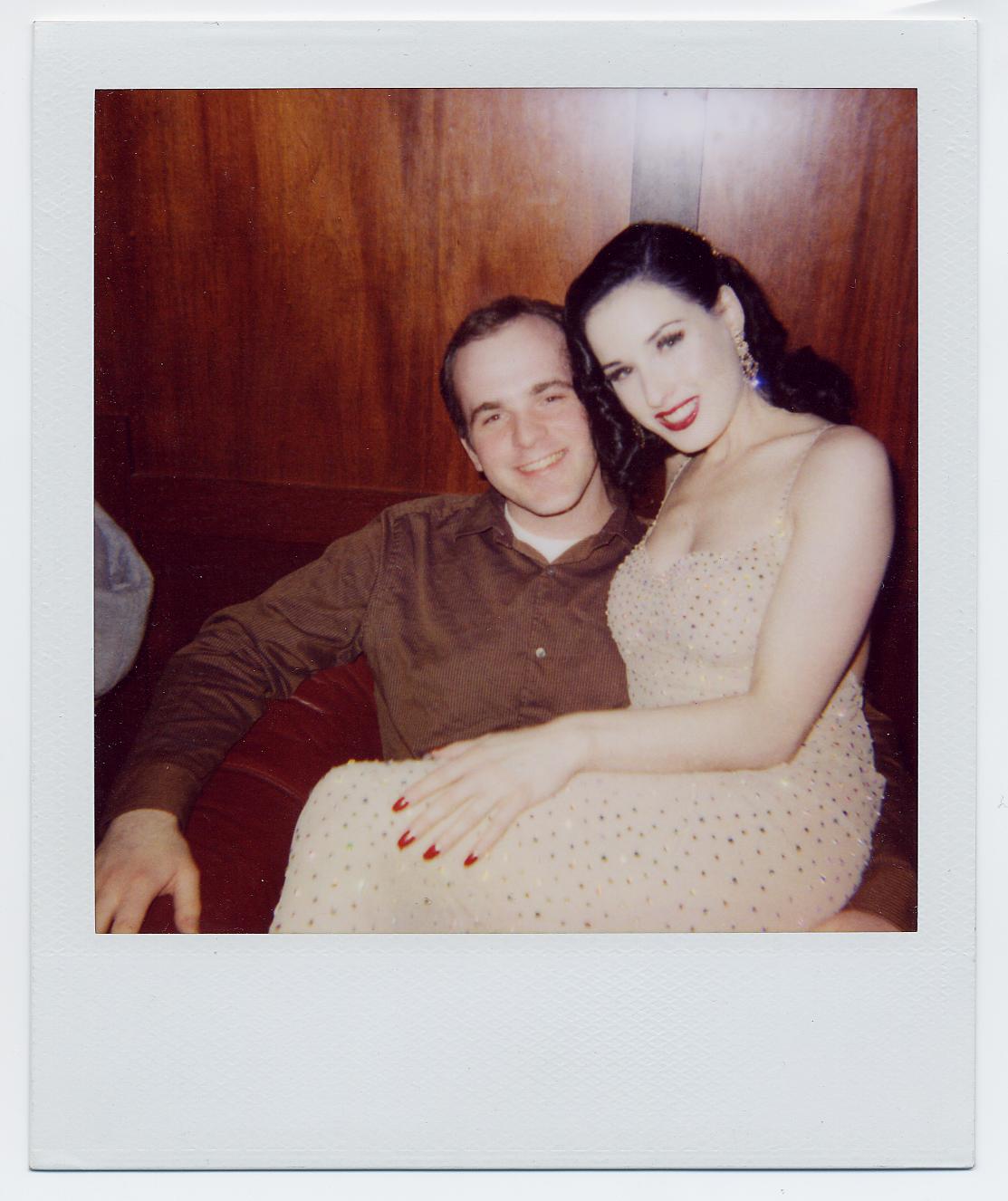In this photographic image set indoors, a young white woman with dark hair cascading past her shoulders, adorned with red lipstick and red earrings, sits on the lap of a young white man. She wears a champagne-colored evening gown embellished with silver rhinestones, with her right hand resting delicately on her leg, showcasing red fingernail polish. The man, dressed in a dark green shirt, beams warmly, sporting a slight receding hairline and brown hair. His right arm is relaxed, resting on what appears to be a sock. Behind them, the wooden paneling of the setting, possibly a house with dark oak-colored walls, adds a cozy, intimate backdrop, emphasizing the personal and affectionate nature of the moment captured.